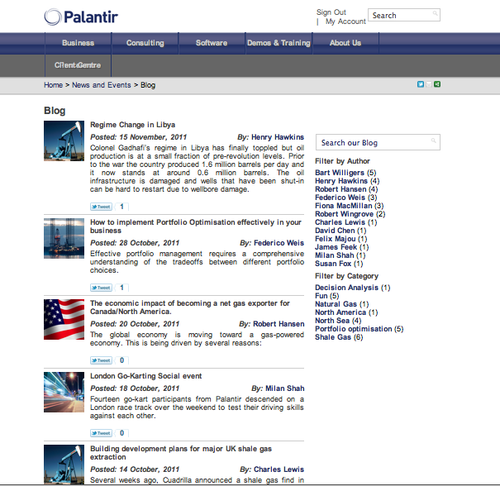In this detailed image of a webpage, the top left corner prominently displays the logo "Palantir." On the top right are various account management options, including a "Sign Out" button, a "My Account" link, and a search field labeled "Search our blogs, filtered by author." Below these options is the main navigation bar containing links to several sections: Business, Client Center, Consulting, Software, Demos and Training, About Us, Home, News and Events, and Blog.

The blog section features a highlighted post titled "Regime Change in Libya," authored by Henry Hawkins and posted on 15 November 2011. The blog post discusses the aftermath of Colonel Gaddafi's regime in Libya, noting that while Gaddafi’s rule has ended, oil production has significantly dwindled to around 0.6 million barrels per day—down from 1.6 million barrels per day before the revolution. The piece further explains that the nation's oil infrastructure is severely damaged, and restarting the damaged wells could be challenging.

In addition to the featured post, there are four other headline articles visible on the page. The search field at the top right specifies its function as searching the blog content and filtering results by different authors, who are listed below the search field.